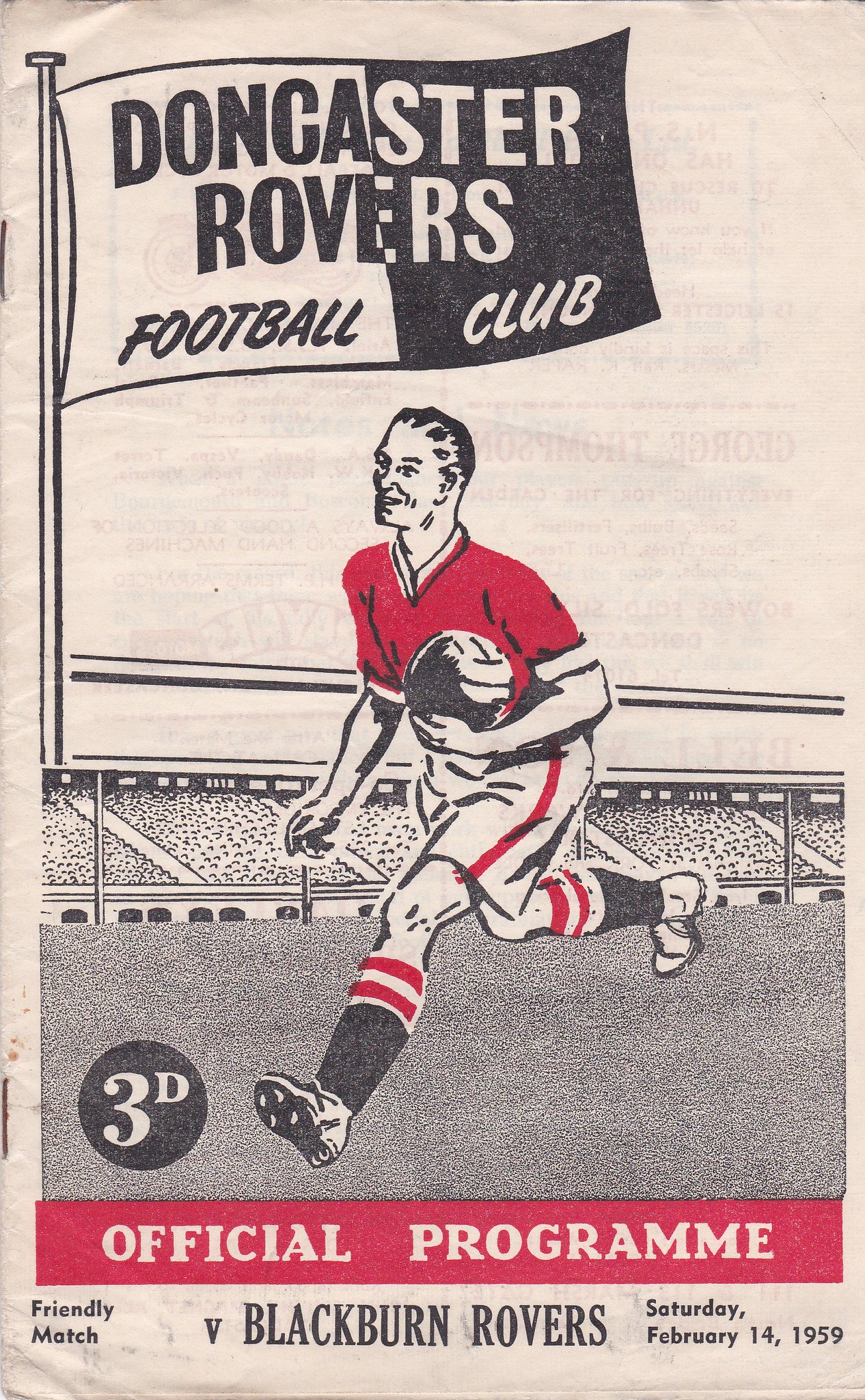This is a color image of an old sports program cover for the Doncaster Rovers Football Club. The primarily black and white illustration, accented with red, features a cartoon sketch of a soccer player holding a soccer ball, running along a soccer field with stadium seats in the background. The player's uniform includes a red soccer jersey, white shorts with red pinstripes, and black socks with red and white stripes around the calf. At the top of the image, a flag with "Doncaster Rovers Football Club" written on it flutters on a flagpole. The program's price, "3D," is indicated above the text. Below the drawing, it states "Official Program," "Friendly Match," "The Blackburn Rovers," and the date: "Saturday, February 14th, 1959."